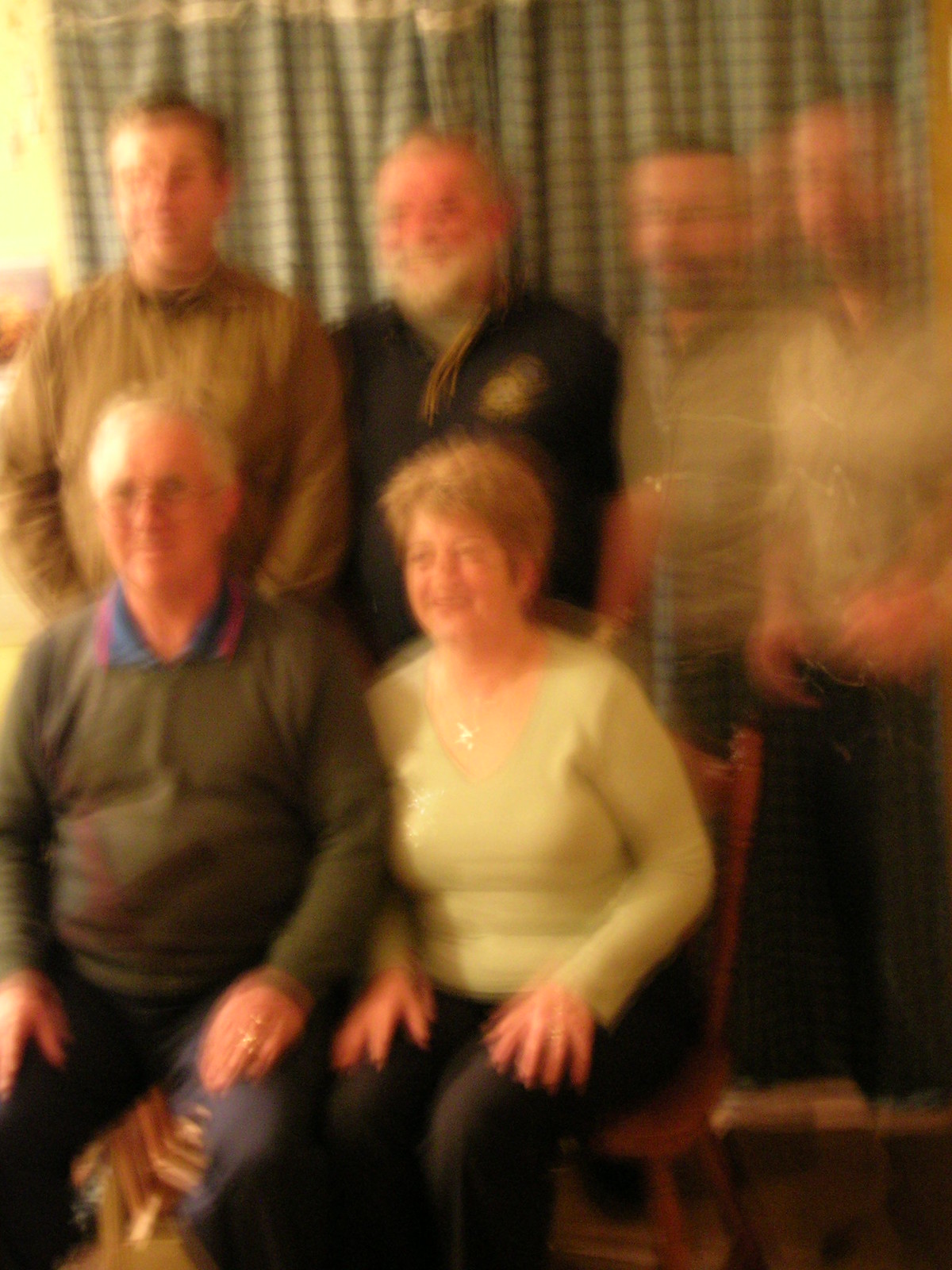This is a slightly blurry family photograph that captures a heartwarming moment. Four men stand in a row behind a curtain, forming a backdrop for the seated elderly couple. The woman, with her short hair styled neatly, is beaming with a warm smile. She is dressed in a light-colored, long-sleeved knit shirt with a v-neck, adorned with a simple yet elegant gold necklace. Her hands rest gently on her thighs, clad in black pants. She is seated comfortably on a brown wooden kitchen chair. Beside her, an elderly man, also smiling, wears glasses and has balding white hair. He is dressed in a green sweater over a collared shirt, paired with dark pants. His hands, like those of his companion, rest on his thighs, exuding a sense of tranquility and happiness.